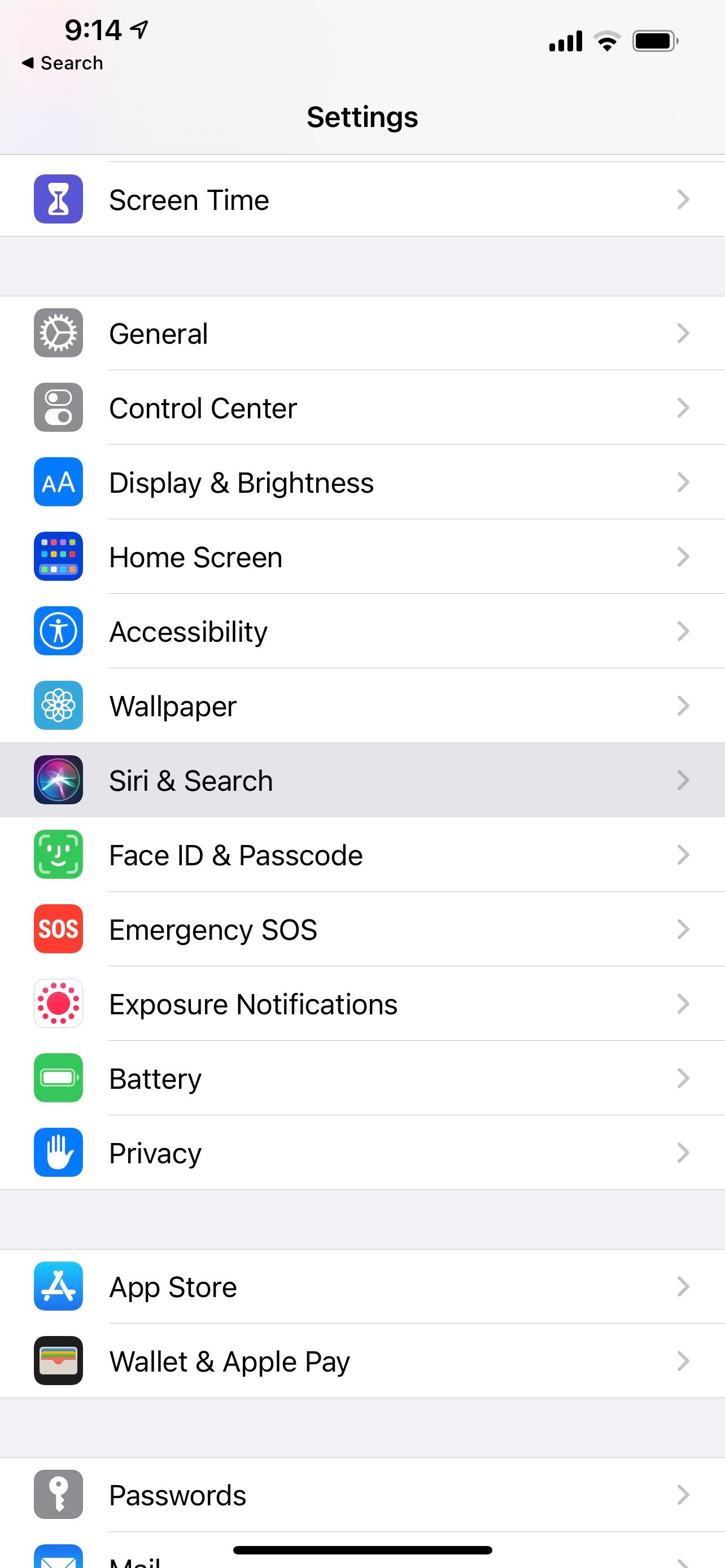The image is a distorted view of an iPhone's settings screen, appearing as if it has been resized and squished, resulting in slightly blurry and disproportionate text. The layout, viewed from an upward angle, gives an impression of protruding towards the viewer. At the top left corner, the screen displays the time as 9:14, alongside four LTE bars, three Wi-Fi bars, and a nearly full battery icon. The title "Settings" is prominently featured at the top.

Below the title, various settings options are listed sequentially with right-pointing arrows next to them, indicating sub-menus. The options are as follows: "Screen Time," "General," "Control Center," "Display & Brightness," "Home Screen," "Accessibility," "Wallpaper," "Siri & Search" (which is highlighted in gray), "Face ID & Passcode," "Emergency SOS," "Exposure Notifications," "Battery," and "Privacy." 

Subsequently, there is a section break followed by options for "App Store" and "Wallet & Apple Pay." Another section at the bottom lists "Passwords" and "Mail," although this part appears to be slightly cut off. Each option is accompanied by its respective icon, and the "Screen Time" option is distinctly separated from the "General" option by a gray rectangle divider, emphasizing its section on the page.